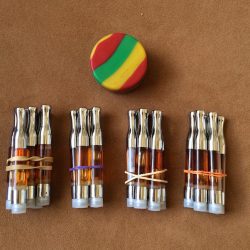This close-up photograph captures a collection of small cylindrical objects resembling cartridges or vape pens, placed on a chocolate brown table. Each cartridge features a silver, metal-like top that tapers into a smaller cylinder, a clear middle section possibly filled with light brown liquid or possessing brown-tinted glass, and a silver bottom capped with silicone. The cartridges are organized into four bundles, each consisting of five or six units, and are secured with rubber bands in various colors: beige, purple, tan, and orange. Positioned above the cartridges is a circular, puck-like object adorned with stripes in yellow, red, green, yellow, and red, resting flat on the table. The reflective surfaces and detailed elements suggest a well-organized arrangement, although the specific function of these items remains ambiguous.